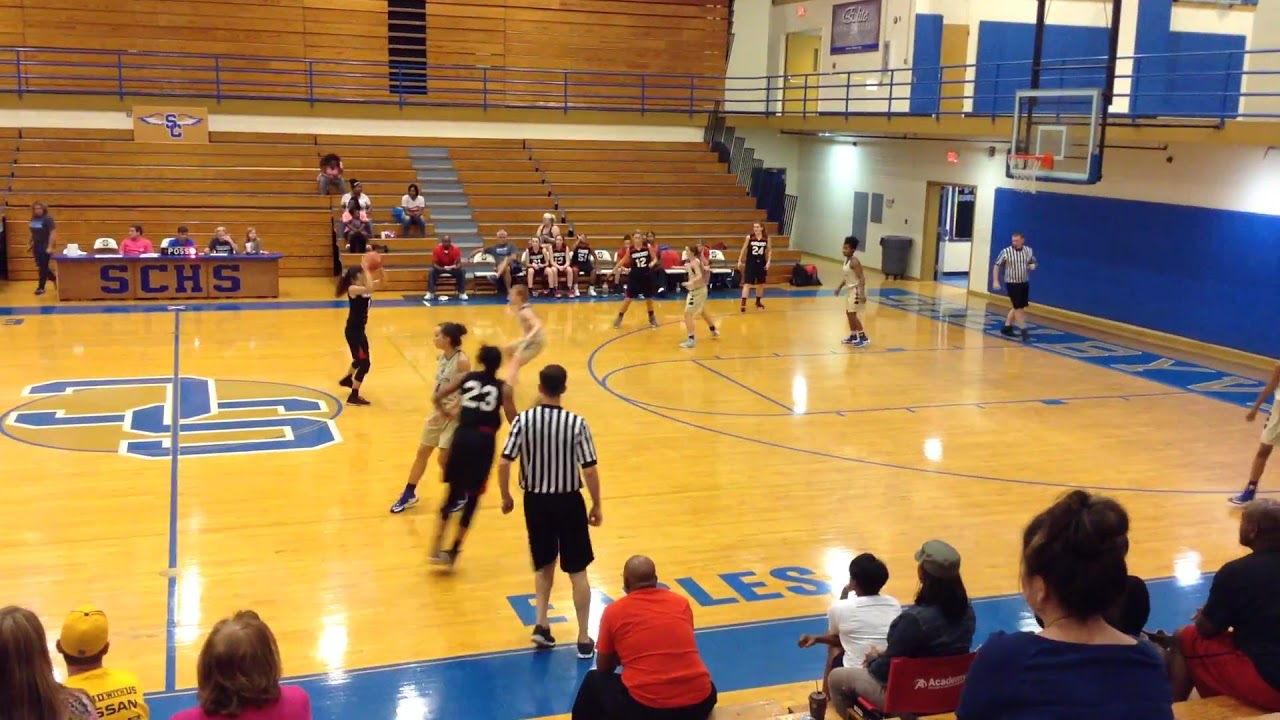The photograph captures an indoor high school girls' basketball game in a brightly lit gym. The gym's floor is a light brown wood, polished to a high shine, with blue accents around the edges. The view appears to be from a spectator's vantage point, slightly elevated in the bleachers, looking down at the court. Two teams are captured mid-action, one in black uniforms with white letters and the other in beige uniforms. The referees are positioned on the court, one with his back to the camera and another to the right. On the opposite side of the court, a table displays "SCHS" in blue, indicating the school's initials, with a few people seated behind it. There are sparsely populated bleachers on both sides, with more spectators visible closer to the camera watching intently. In the background, an exit and a trash can can be seen on the right, along with an upper-level railing that suggests an indoor walking area above. One player is about to throw the ball to a teammate as another player rushes towards her, capturing a dynamic moment of the game.